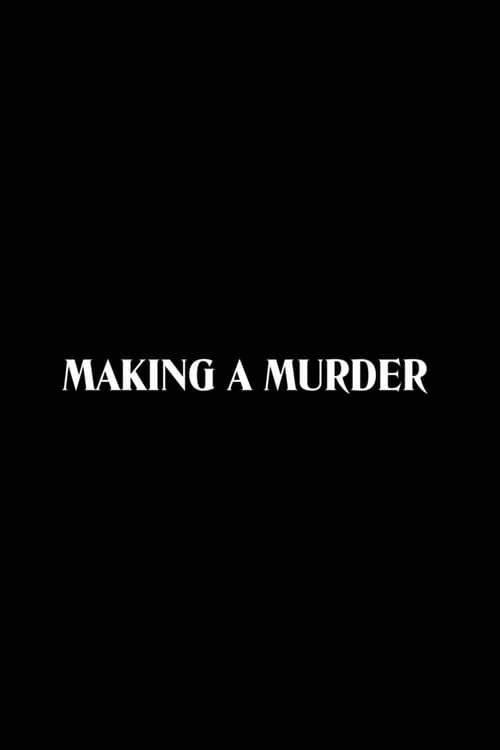The image is a tall, vertical black rectangle, significantly longer than it is wide, devoid of any borders or additional objects. Positioned centrally within this stark, void-like background are three words in bold, capitalized white font: "Making a Murder." The lettering appears somewhat formal yet has a loud and potentially sinister aesthetic, likely intensified by the word "murder." The text occupies minimal space, reinforcing the simplicity and emptiness surrounding it. The visual could serve as a cover of a book, a frame from a presentation, or more plausibly, a promotional poster due to its minimalist and impactful design.